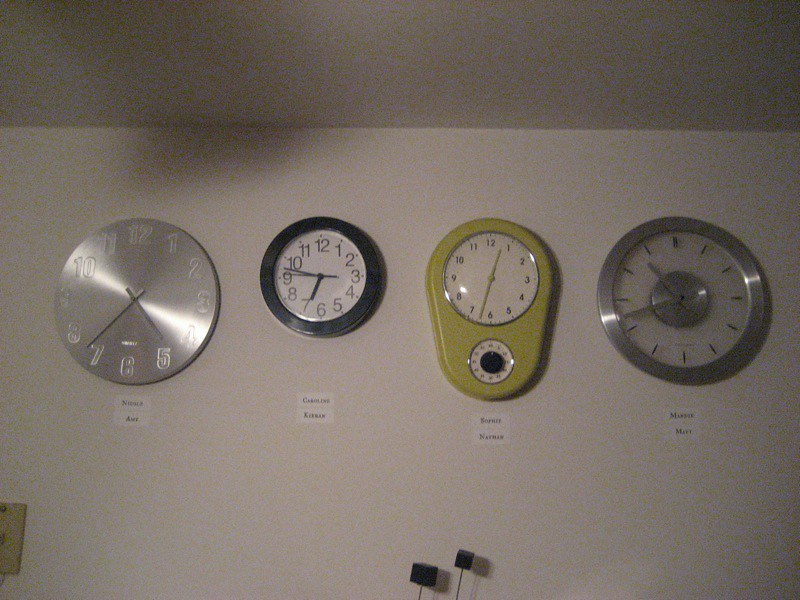The indoor photograph depicts a wall near the ceiling adorned with four horizontally-aligned clocks, each indicating a different time zone. Starting from the left, the first clock is a sleek silver design with embossed white numerals from one to twelve. It features two black hands and shows the time as approximately 4:36. Directly adjacent is a smaller clock with a black rim and a white face, numerically marked from one to twelve, displaying the time as 6:47. The third clock is distinctive with its greenish, potentially dual-faced design. It has black numerals on a white background, hands showing about 12:32. Lastly, the fourth clock has a minimalistic silver rim with dash marks instead of numbers, and two silver hands pointing to around 10:42. Below each clock, there are labels with unreadable text, possibly denoting the corresponding time zones. The muted variety in clock designs and times suggests a visual representation of different global time zones.